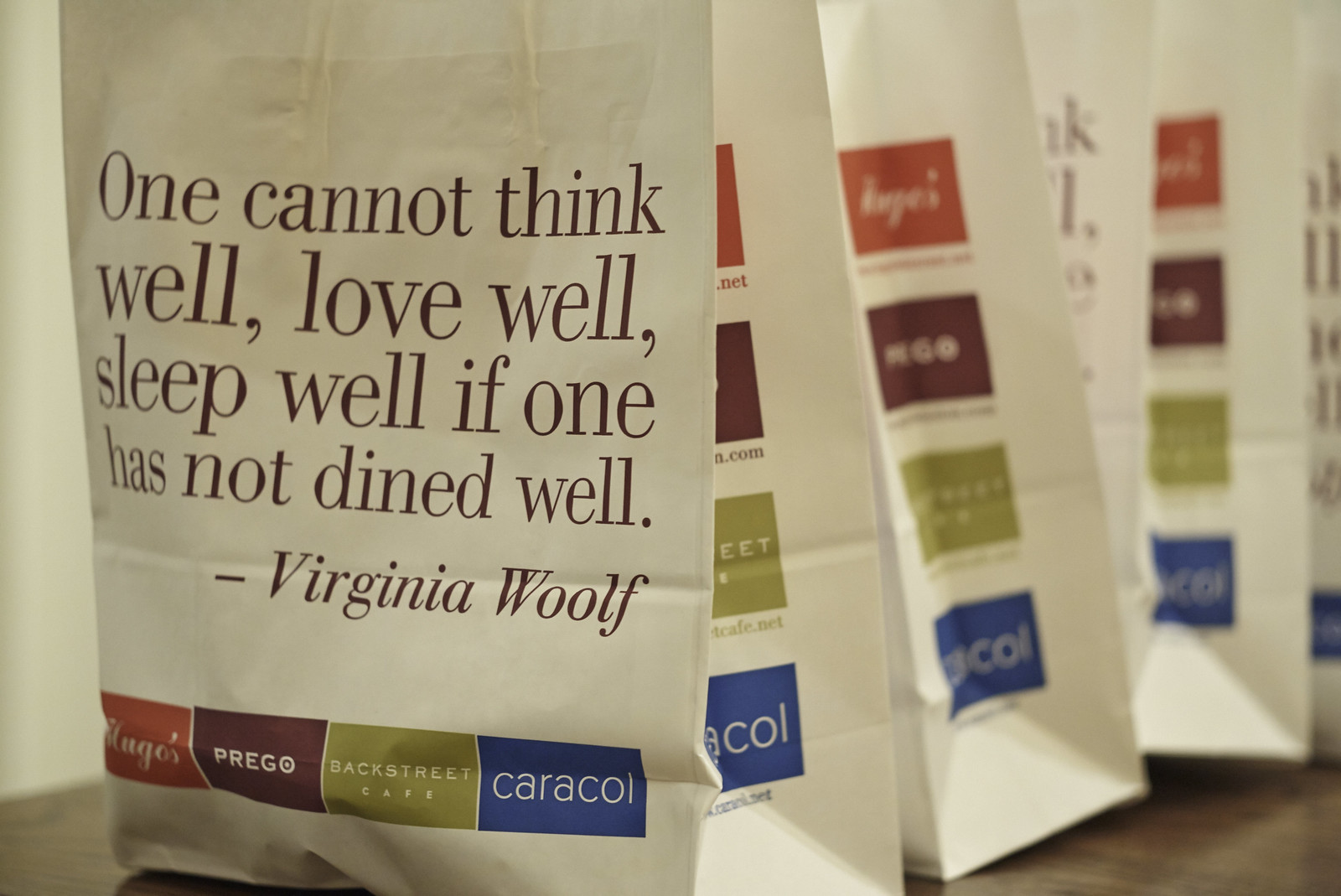This photograph captures a row of approximately four open white paper gift bags, neatly aligned on a brown wooden table. Each bag prominently features a quote in maroon-colored ink that reads, "One cannot think well, love well, sleep well, if one has not dined well" - attributed to Virginia Woolf. Below the quote, the bottom of each bag is adorned with logos of four different sponsors represented in differently colored squares: red for Hugo's, maroon for Prego, lime green for Backstreet Cafe, and blue for Caracol. The same logos appear on the sides of the bags along with a web address: "www.Flydreamers.com". These bags evoke the impression of being ready for either a special event or takeout food pickup.